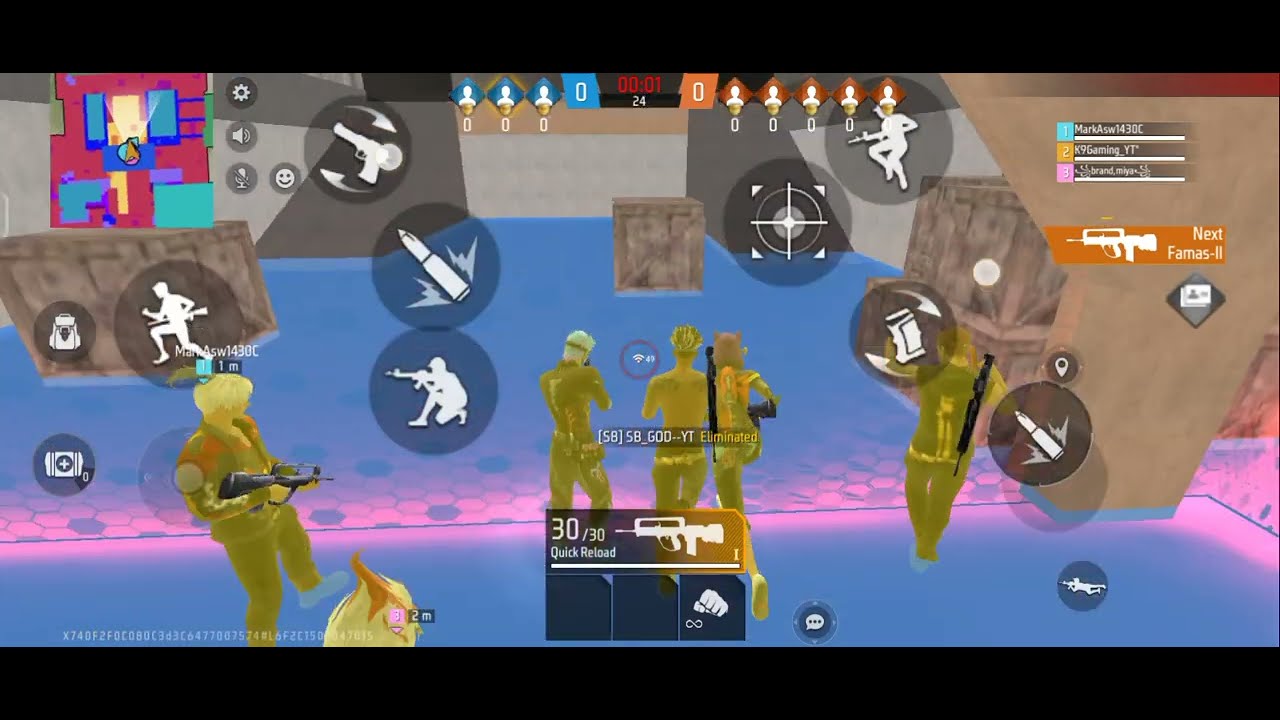The image is a detailed screenshot from a video game, showcasing a scene that appears to be from a militaristic shooter game. At the center of the image, three humanoid characters with their backs facing the viewer are highlighted, all rendered with a golden, translucent hue, possibly due to an active menu screen. Flanking them on the left and right sides are two more similarly designed characters, each holding automatic weapons. The bottom center of the screen displays a weapon selection menu, showing an automatic assault rifle with an ammo count of 30/30, and an icon of a fist, suggesting melee options.

The screen is filled with various game HUD (Heads-Up Display) elements: in the top left corner, a mini-map is visible, which helps the player navigate the environment. Below the mini-map, there are several icons, including a crouching person with a gun, a circle with a plus sign (likely indicating health), and another indicating a bag, which could signify inventory or gear. Additional icons like a bullet and crosshairs are peppered across the screen, enhancing the tactical feel of the game. The top right corner displays player rankings with usernames, labeled 1, 2, and 3.

The environment portrays wood crates and a ramp on the left side, which could offer strategic cover or contain supplies, hinting at potential gameplay mechanics involving exploration and inventory management. The combination of these elements suggests a deeply immersive and interactive gaming experience.